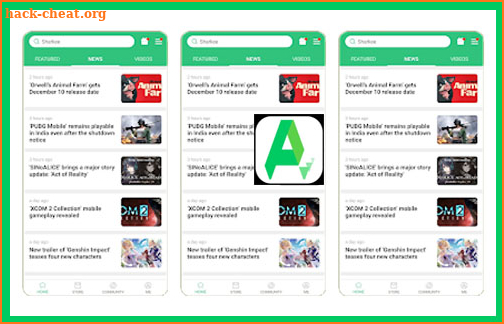The image showcases a visually engaging website primarily designed for a cellular program. At the top right corner of the website, a distinct border marked by contrasting colors highlights the background. Various icons are strategically dispersed across the middle section of the page, presenting an array of shapes accompanied by text. The website displays a diverse palette of colors, creating a visually stimulating experience.

Notifications are prominently positioned throughout the page, appearing at the top, middle, left, and right sections. Numerous images populate the website, each featuring unique colors, text, and shading to emphasize their significance. The overall layout is medium-sized, ensuring ease of access and navigation. The structured design facilitates quick information retrieval, allowing users to find desired content effortlessly and efficiently.